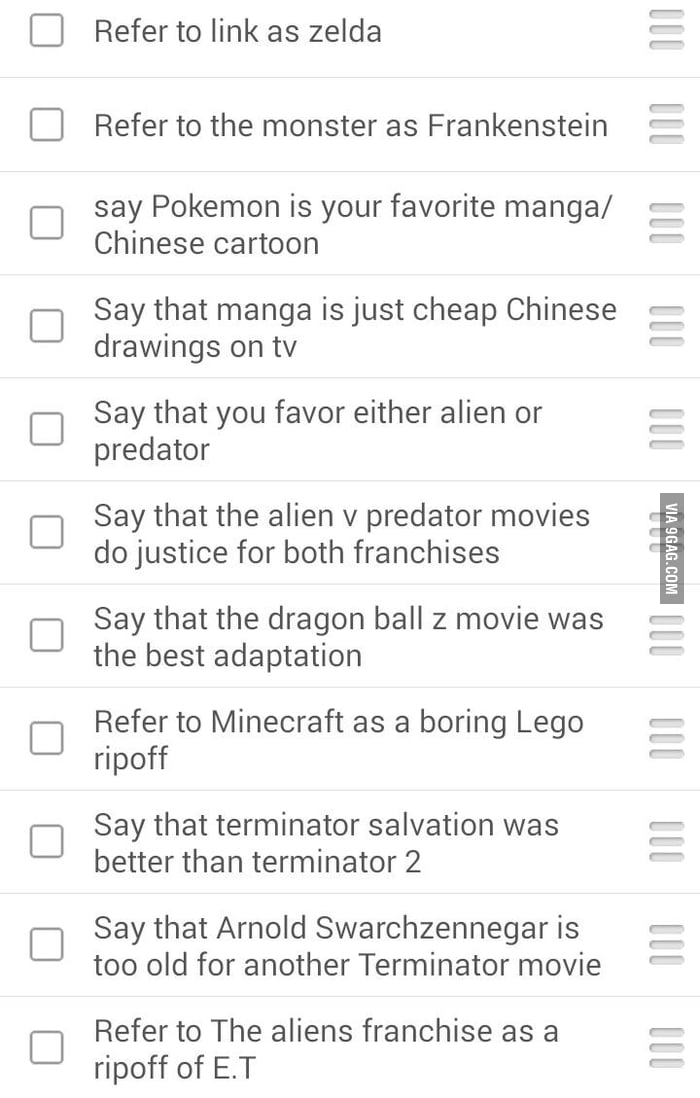The image portrays a list with several references, each accompanied by a checkbox for marking completion. The references list includes the following points, each flanked by checkboxes on the left and three horizontal lines on the right:

1. Refer to the character Link as "Zelda".
2. Call the monster Frankenstein.
3. Describe Pokémon as your favorite manga, noting it as a Chinese cartoon or Japanese comic, with an associated checkbox.
4. Refer to manga as cheap Chinese drawings or simply cheap drawings on TV.
5. State your preference for either Alien or Predator.
6. Claim the Alien vs. Predator movies as representing both franchises.
7. Describe Dragon Ball Z movies as the best adaptations.
8. Mention Minecraft as a boring LEGO ripoff.
9. Say that the first Terminator movie was better than Terminator 2.
10. Argue that Arnold Schwarzenegger is too old for another Terminator movie.
11. Refer to the Aliens franchise as a ripoff of E.T.

The checkboxes next to each statement visually indicate whether each reference has been acknowledged or agreed upon.